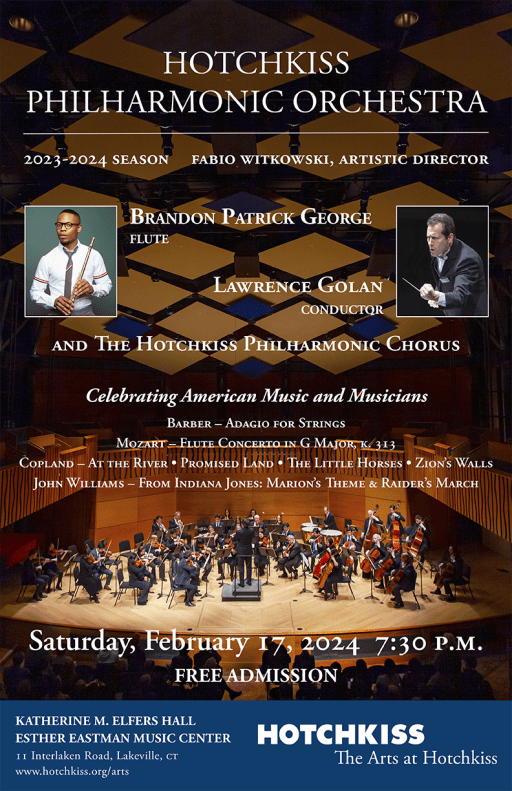The flyer for the Hotchkiss Philharmonic Orchestra showcases a vivid photograph of the orchestra mid-performance inside a sophisticated and brightly lit wooden auditorium. The roof of the auditorium features an intricate design of alternating orange and blue geometric squares, giving a visually striking backdrop to the stage. The stage is filled with musicians playing a variety of instruments, including cellos, violas, violins, and drums, all under the baton of the conductor. In front of the stage, a full audience can be seen, engrossed in the performance. The top of the flyer prominently displays the text "Hotchkiss Philharmonic Orchestra" in white font, outlining the 2023-2024 season. Additional details include the year of the season, the artistic director, and highlighted performers, such as the flutist and the conductor. The flyer also lists the themes of the performances and provides specifics about the acts they will interpret. At the bottom, essential event information is presented: "Saturday, February 17, 2024, 7:30 p.m., free admission." The very bottom of the flyer features a blue rectangle with the text "Hotchkiss, the art at Hotchkiss," followed by an address and website.